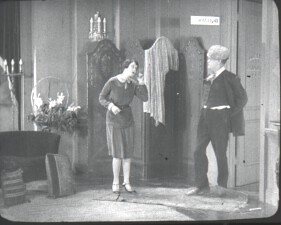This black-and-white image, reminiscent of an early 20th-century movie still or theater play scene, features antique decor that evokes a vintage aesthetic from the 1940s or 1950s. At the center stands a woman dressed in a long-sleeved, vintage-styled dress with a period-specific haircut. She appears engaged in conversation, her head tilted slightly to the left, addressing a man positioned on the right side of the frame. The man is clad in black pants, a shirt, and a long black jacket, and he wears a distinctive fuzzy hat. Behind him, an open door adds depth to the scene. To the left of the woman, a wardrobe is visible with a candelabra adorned with candles sitting atop it. Additionally, there are flowers, rugs, and cushions around the room, enriching the set with an antique ambiance. The detailed decorations, including another candelabra and numerous candles on a table, further enhance the classic, bygone era feel of the photograph.